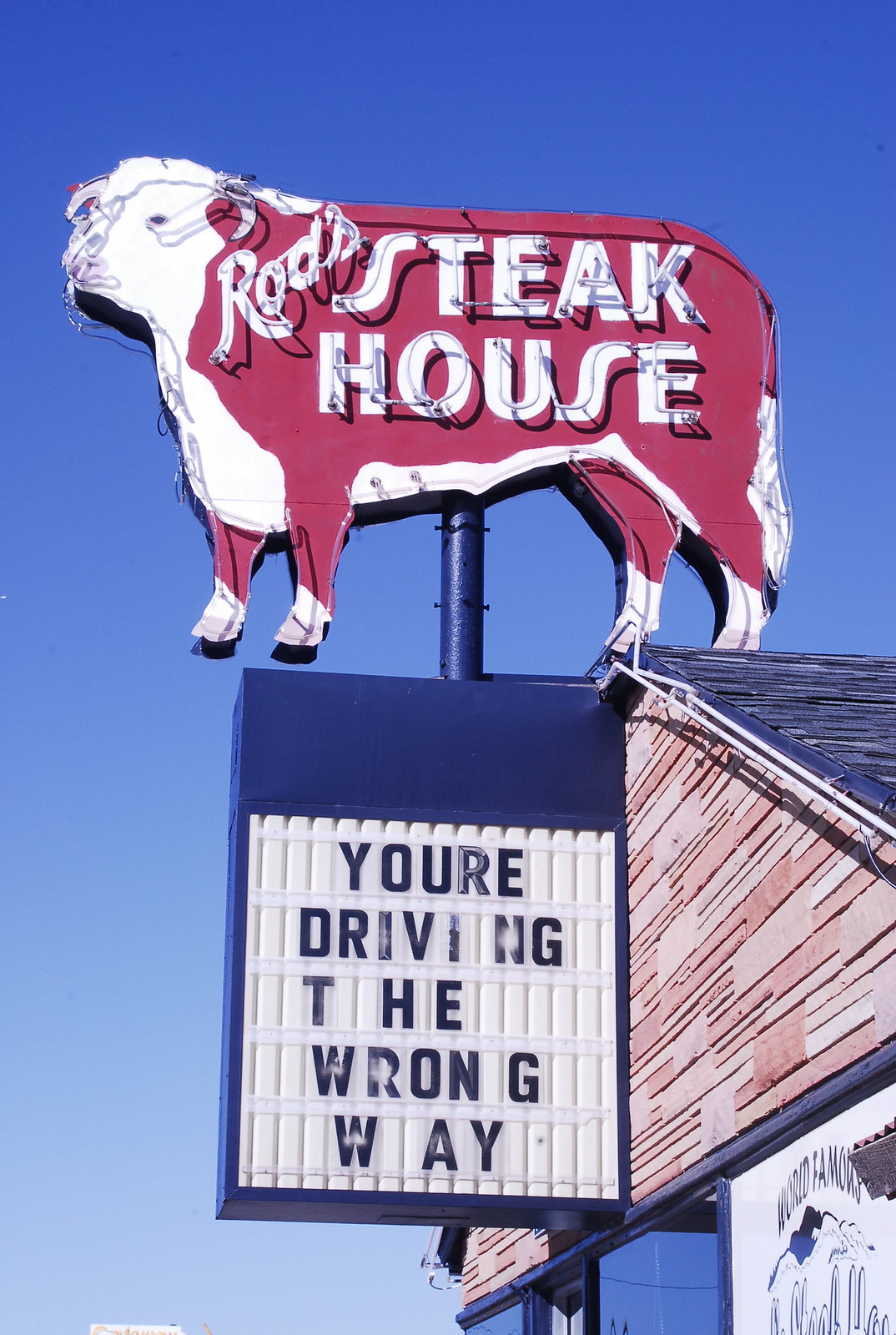This photograph captures the front of Rod's Steakhouse, looking up at a prominent sign against a completely blue sky. The sign is mounted on a pole attached to the end gable of the restaurant's pitched roof. The roof features red and pinkish shingles, while the building itself is painted blue.

At the top of the sign, there is a red and white steer, with a white head, belly, and underside, and red covering the rest of its body. Across the steer's back and side, the words "Rod's Steakhouse" are written in white, appearing to be neon lights that would illuminate at night. Below this, the sign has a rectangular section with a blue border and a white background which displays the message “You’re driving the wrong way” in black letters. Notably, the first letters of "the" and "way" are spaced slightly further apart than the rest.

This detailed setup conveys both the unique charm of the steakhouse's signage and its assertive roadside alert, emphasizing its welcoming yet quirky character.